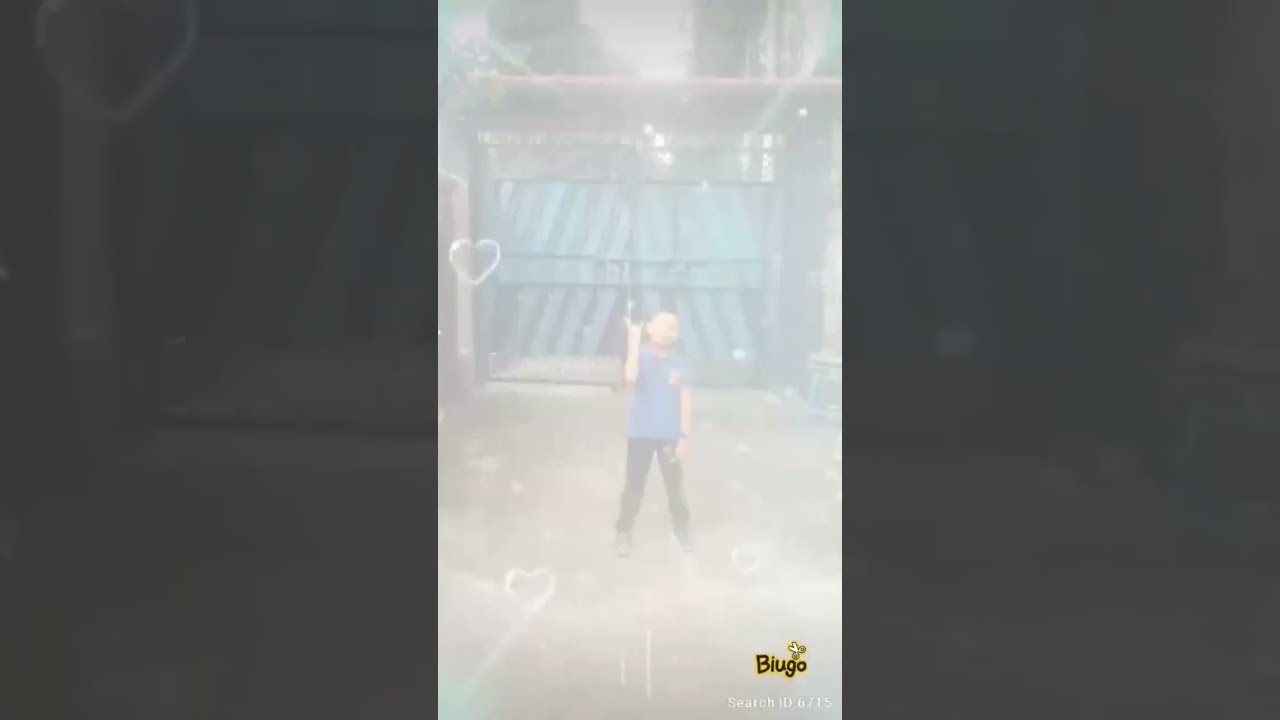In this image, a young child stands centered against a background that includes a textured wall with shades of light and dark blue and possibly a large green metal gate. The child is wearing a blue (possibly aqua-colored) T-shirt and black pants, striking a pose with their left hand raised in a gesture resembling "metal spikes." The entire image is veiled with a hazy, white film and appears softly blurred, potentially from a filter or smokiness, accentuated with heart shapes that contribute to the overall soft and indistinct quality. The ground under the child seems to be concrete, adding to the industrial feel of the setting. In the bottom right corner, there is black text with a yellow outline that reads "B-I-U-G-O," accompanied by an icon of scissors and the additional text "Search ID 6715."